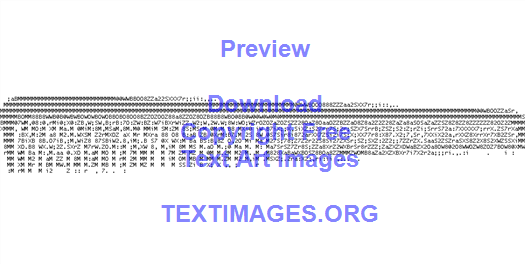The image is a text art representation of a comb, made up of small ASCII characters like letters and numbers. It originates from a website called textimages.org. The image prominently features a blue watermark that reads "PREVIEW," followed by "DOWNLOAD," "COPYRIGHT FREE," and "TEXT ART IMAGES." These texts are stacked in blue letters and conclude with "TEXTIMAGES.ORG" in all caps at the bottom. The background is entirely white, creating a stark contrast with the black ASCII characters forming the comb. The top-left portion of the comb clearly shows the bristles, while the rest of the design becomes less distinct as the characters merge together. The intricate text art demonstrates an art form popular during the early internet days, where keyboard characters were used to create visual images.